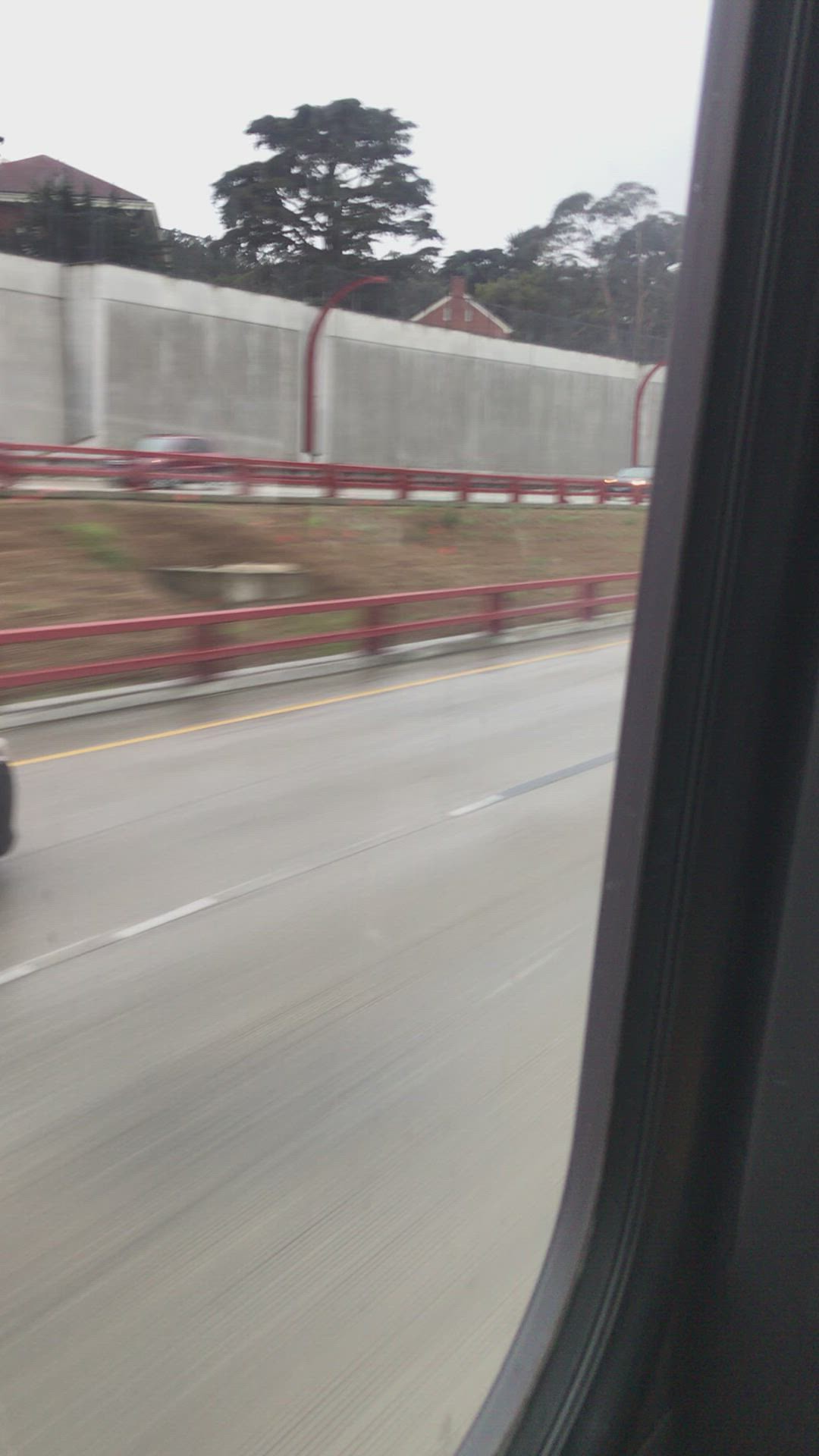This image is a photograph taken from inside a moving vehicle, possibly a bus or truck, capturing a street scene through a large, rounded side window. The window frame and molding trim are visible on the right-hand side, indicating the photo was taken from inside the vehicle. The road is discernible at the bottom of the image, made of gray concrete cement, and marked with dotted white lane dividers and a yellow stripe along the outer lane, typical of a freeway. A red-painted guardrail borders the road, beyond which lies a strip of green grass. Further up, there is another red guardrail, after which the ground slopes upward to a higher level where more traffic is visible. A large concrete retaining wall runs parallel to the roadway, and in the background, the top of an A-frame roofed house is visible along with another building in the upper left corner. The sky appears gray and overcast, adding to the overall atmosphere of the scene. The image captures some motion blur but remains generally clear, highlighting the multi-layered layout of the streets and structures.